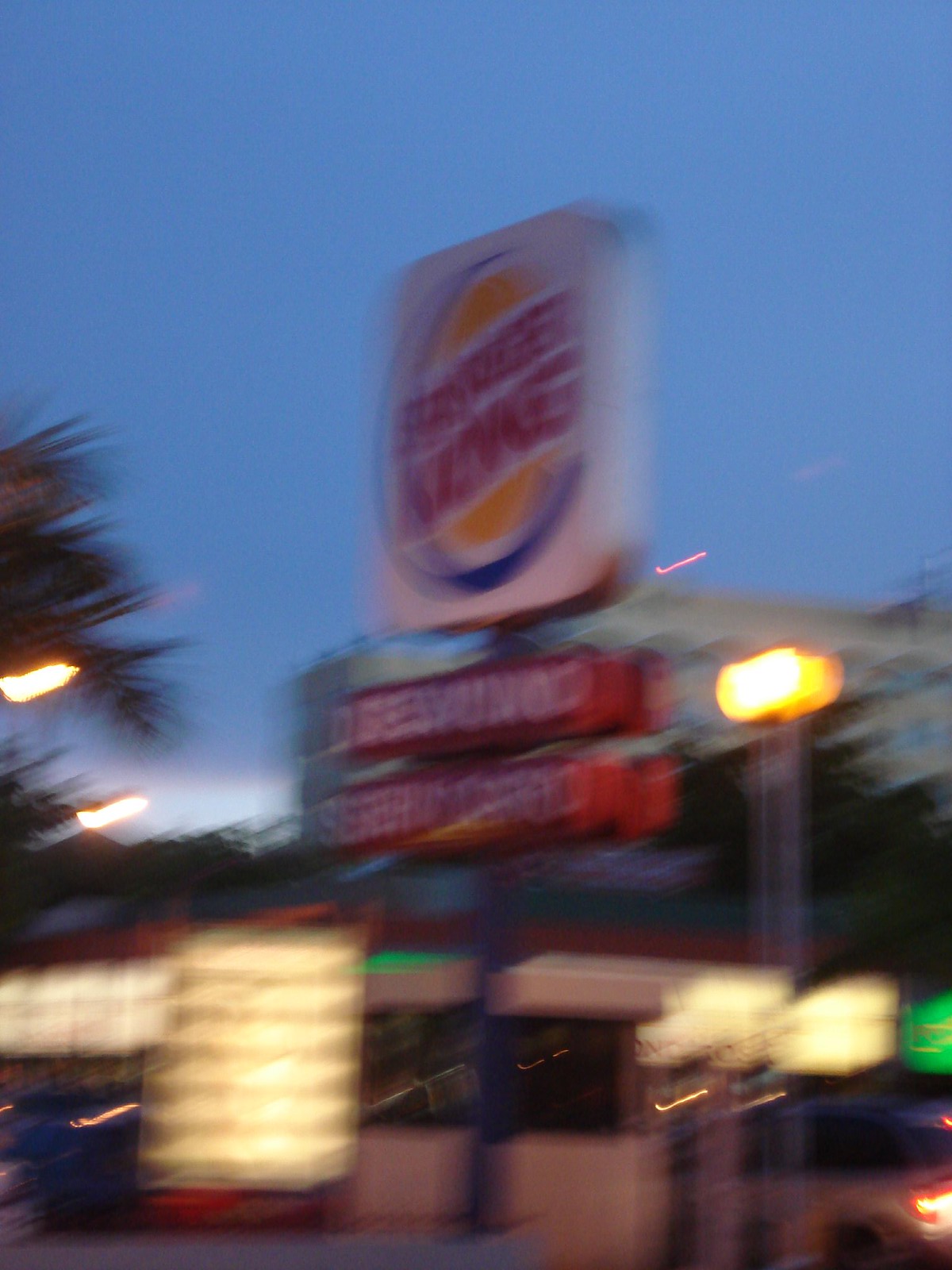In this blurred, nighttime photograph, the viewer can discern a prominently featured Burger King sign atop a dark-colored metal post. The sign displays the familiar circular blue and yellow Burger King logo with red lettering, though it is not internally illuminated. Positioned below the main sign are two red rectangular signs with illegible white text. The scene is bathed in the sodium yellow glow of nearby streetlights, suggesting the image was captured either at twilight or after dark. A deepening blue sky forms the backdrop, with tree foliage visible on the left side, adding a touch of nature to the urban setting. The bottom of the image faintly reveals what appears to be a brightly lit gas station, contributing to the overall illumination in the area. Additionally, a blurry object in the lower right corner hints at a moving vehicle, possibly indicating that this photograph was taken in transit.